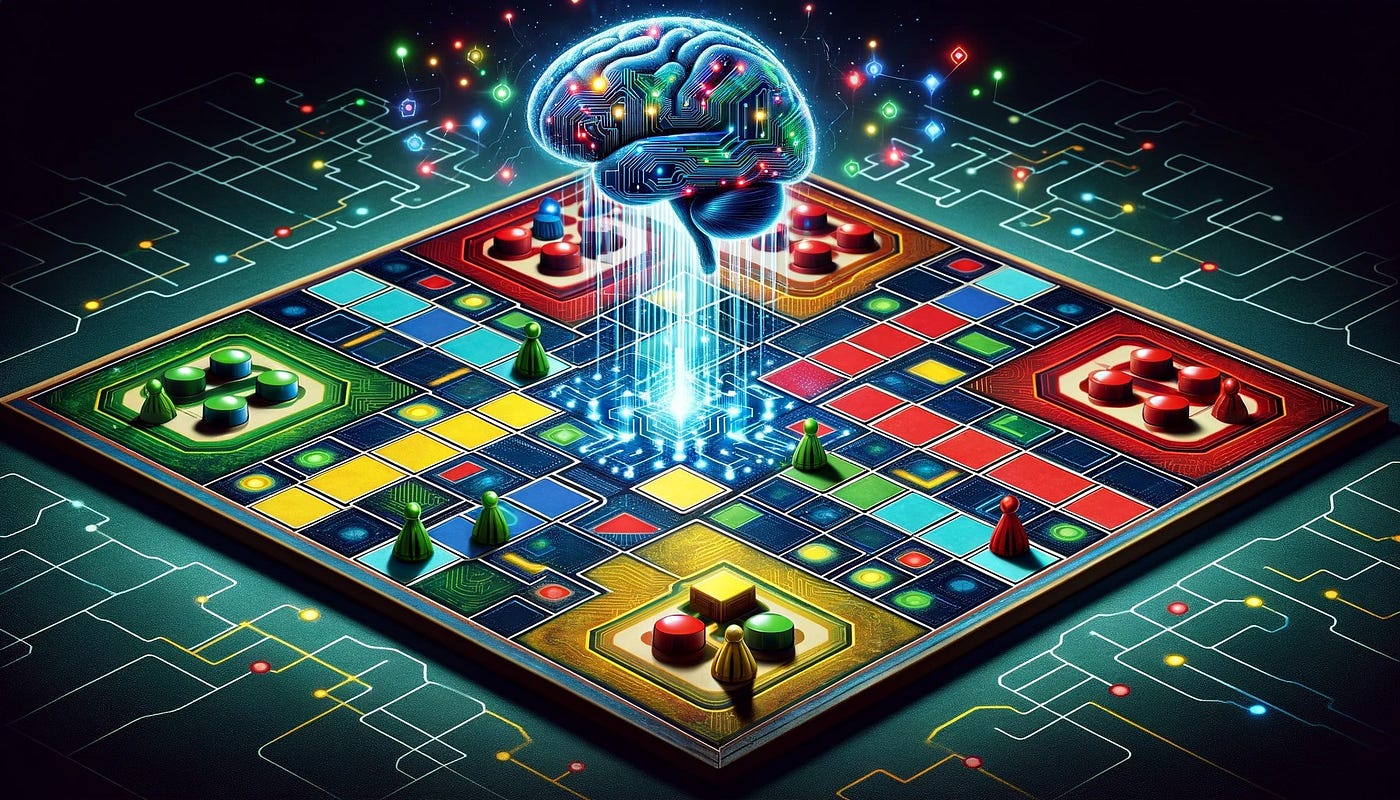This detailed 3D rendering depicts a futuristic board game reminiscent of Parcheesi, with a digitized, AI-created aesthetic. Central to the image is a cyan-colored human brain, adorned with a spectrum of gemstone-like lights in red, yellow, green, and blue, and surrounded by a futuristic computerized chip design. The brain floats above the board, casting a luminous beam downwards, illuminating the entire board.

In each of the board's corners are distinct home bases: green in the left corner with four green circles and a green pawn; red on the right with four red cylinders and a red pawn; yellow at the bottom front with one yellow square, one red cylinder, one green cylinder, and one yellow pawn; and an orange-yellow base in the back corner with four red cylinders. From these bases, various colored game pieces resembling Sorry pieces move across the board. Notably, two green pieces have advanced towards the center, accompanied by a scattering of red, yellow, and green pawns making their way along the circuit-like pathways.

Edge to edge, the board is detailed with intricate circuitry lines in multiple colors—blues, yellows, reds—highlighting the high-tech theme. The center of the board glows brightly from the brain's light, while the peripheries remain darker, emphasizing the illuminated central action. The board itself is elevated in design, encircled by a solid black border that contrasts sharply with the vibrant interior, creating a visually striking and immersive gaming experience.